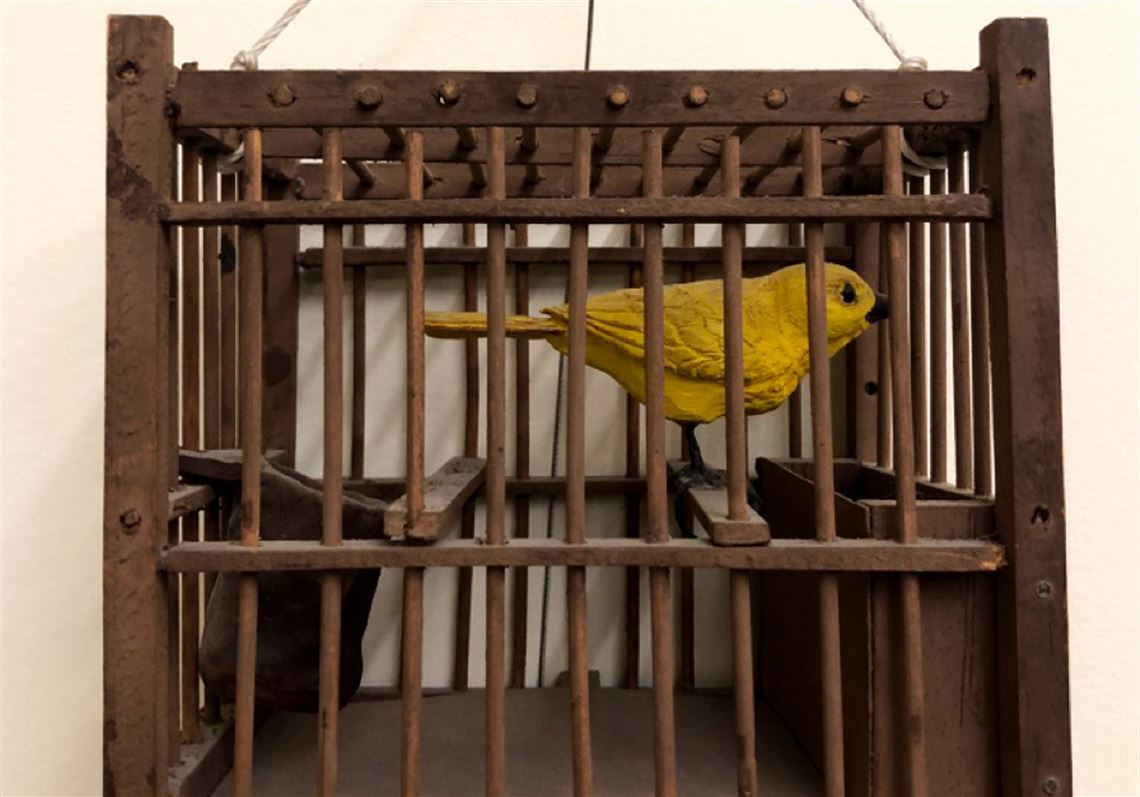The image features a small, yellow parakeet-like bird inside a brown or rust-colored cage that may be crafted from wood or iron. The cage appears to be handmade, as indicated by its slightly uneven bars, and is suspended by thin, white strings or ropes. The background consists of a plain white or tan wall. The bird itself has dark, bulging eyes and a dark beak, with detailed features suggesting it could be a wooden statue painted to mimic a real bird. Inside the cage, there are two containers: a rectangular box on the right and a circular bag or tray on the left, likely intended to resemble bird feeders. The base of the cage is flat and brown, complementing the rustic aesthetic of the scene.